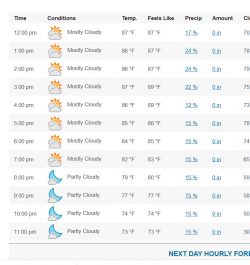This image is a cropped screenshot showcasing an hourly weather forecast. The snapshot, shaped as a square, does not reveal the source website. At the top, several columns are labeled from left to right: Time, Conditions, Temperature, Feels Like, Precip (for precipitation), and Amount. The name of the last column is partially cut off, showing only the letter 'C'.

On the left-hand side, the times run hourly from 12 p.m. to 11 p.m. Under the Conditions column, from 12 p.m. to 7 p.m., the forecast predicts "Mostly Cloudy," accompanied by an icon depicting two clouds with an orange semicircle representing the sun peeking out. From 8 p.m. to 11 p.m., the forecast changes to "Partly Cloudy," shown by an icon featuring a blue crescent moon and a cloud, indicating nighttime conditions.

The Temperature and Feels Like columns provide varying hourly temperatures, while the Precipitation column details the chances of precipitation and its amount. At the bottom right-hand corner, the words "Next Day Hourly" are visible, with the beginning of the next line reading "FOR" partially cut off.